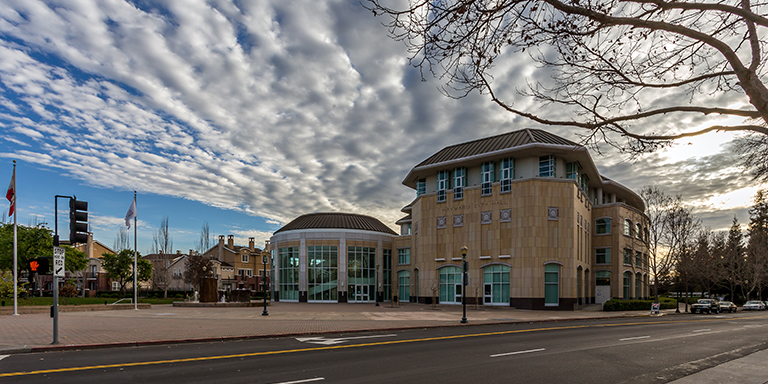This outdoor photograph captures a stately, yellow-stone building that appears to be Harvard City Hall under a bright blue sky scattered with fluffy clouds. The building, primarily constructed with stacked yellow stones for the first three stories, contrasts with a white material used on the fourth level. The structure commands attention with its classic, sophisticated architecture typical of an upper-class East Coast city. To the left of the City Hall stands a unique, round building enveloped in glass windows from floor to roof, likely serving as a pavilion or greenhouse that floods with natural light. 

In the foreground, a road runs adjacent to the building, bordered by a large brick sidewalk. To the right, bare-limbed trees suggest a winter setting, their stark branches silhouetted against the sky. Several flagpoles with low-hanging flags and a streetlight sign punctuate the scene on the far left. The bustling yet serene environment is further complemented by parked cars and additional older-looking buildings in similar architectural styles dotting the background. The vivid detail, enhanced slightly by HDR manipulation, makes the inviting day feel crisp and clear, encapsulating a picturesque slice of Harvard’s urban landscape.